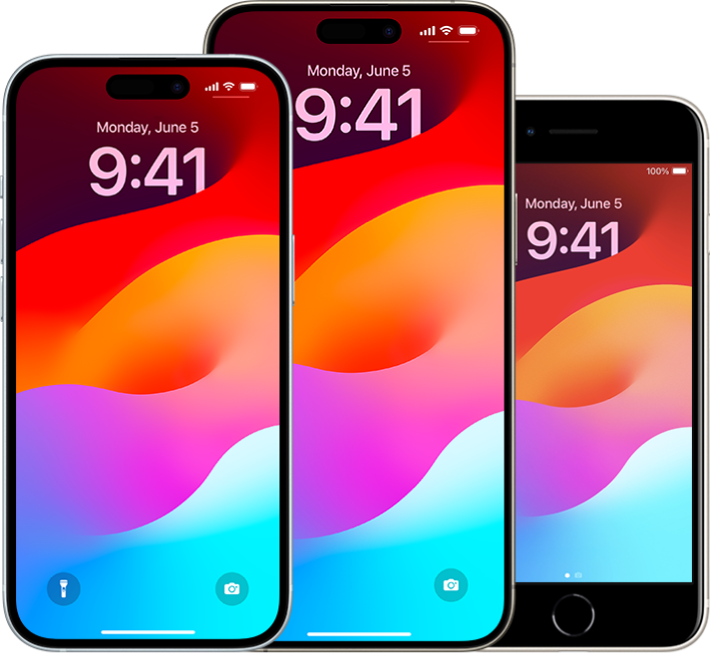The image showcases a set of three iPhones, appearing to be an advertisement for the models. All three phones are displayed against a white background with softly rounded corners, showing identical lock screens. The screens indicate the time as 9:41 AM on Monday, June 5th, and depict fully charged batteries and active Wi-Fi icons. The lock screens feature a vibrant, abstract art motif with swirling colors transitioning from teal blue and magenta to orange, yellow, and red, evoking a lava lamp-like effect. Positioned upright, the middle iPhone is the largest, possibly a plus model, flanked by two smaller models of approximately equal size on its left and right. Each phone's home screen includes icons for a flashlight and a camera at the bottom, and the smaller rightmost model features an additional fingerprint sensor button at its base.